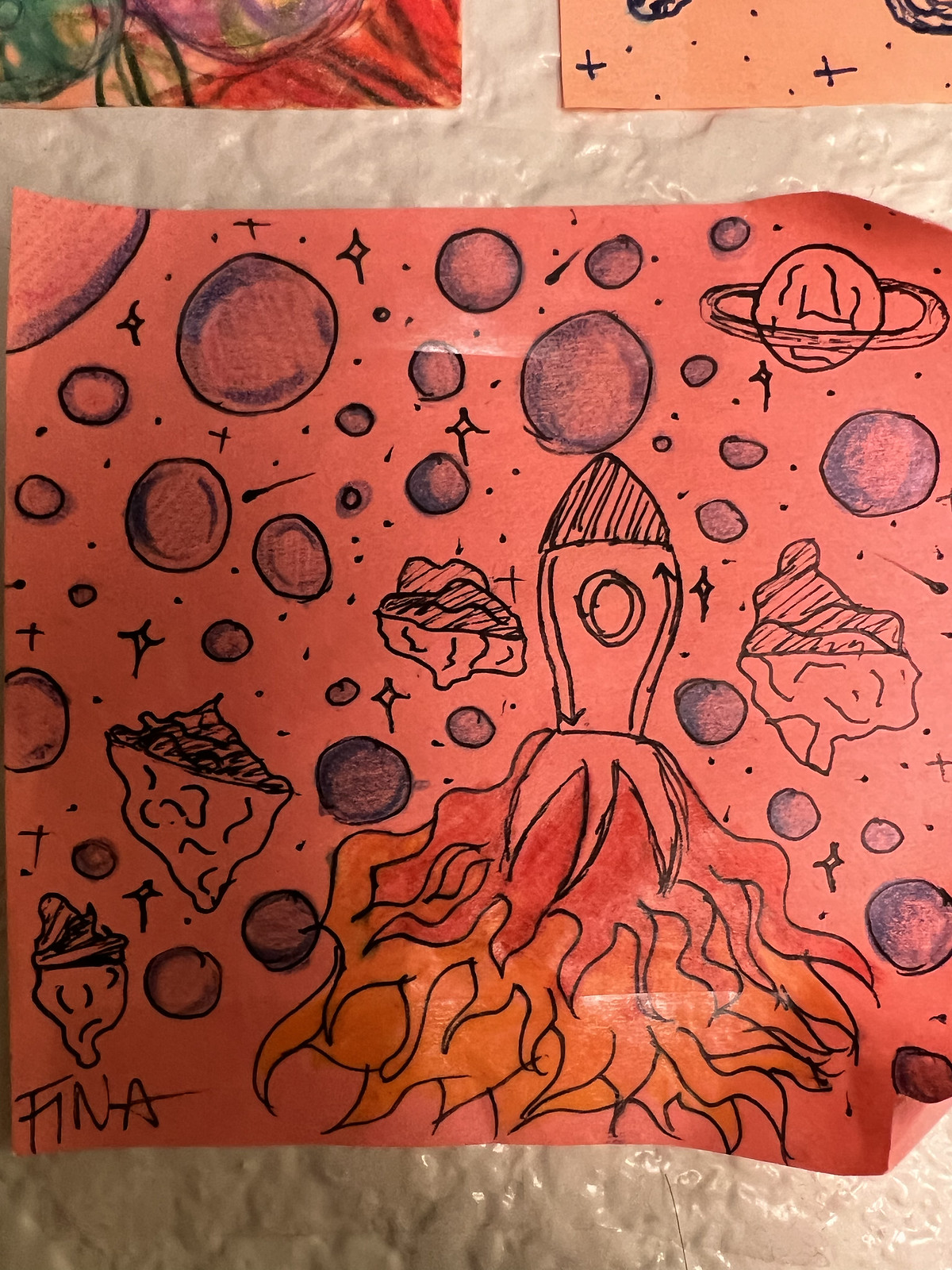A detailed photograph captures a child's bedroom wall, adorned with a dated, textured wood chip wallpaper painted a dark salmon color. Prominently displayed is a large, vertically-oriented drawing, signed "FINA" at the bottom left. The artwork, rendered in black ink on salmon-colored paper, depicts a simple, spoon-shaped rocket amidst a chaotic and imaginative space scene. Red and yellow flames burst out from the rocket's base, surrounded by an array of celestial objects including planets, stars, asteroids, and floating islands with mountains. The upper corners of the image reveal the edges of two additional, partially visible drawings—one in vibrant colors featuring reds, seafoam green, and purples, and the other in simple black marker with plus signs and dots. The scene suggests the vastness of space with its moons, a large planetary body at the top left, a ringed planet at the top right, and various meteorites and shooting stars scattered throughout. The entire arrangement exudes a sense of textured roughness, highlighted by the crinkly, off-white background that mimics the surface of the moon.